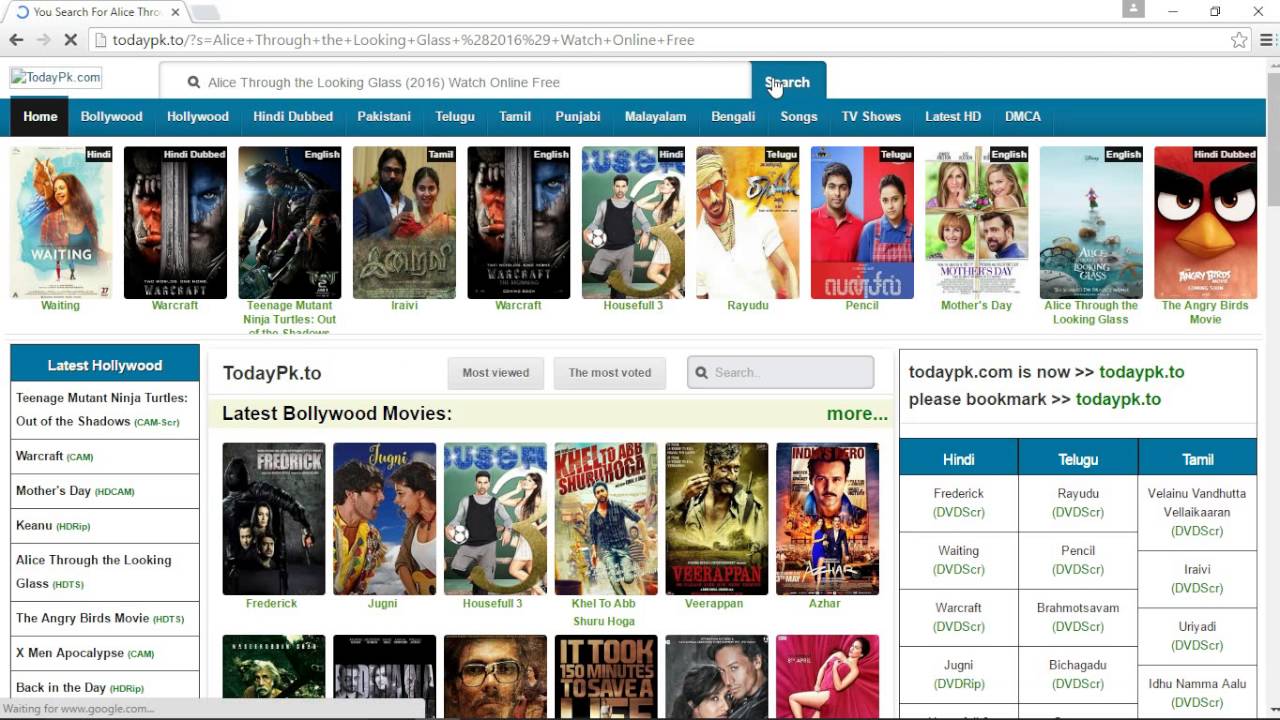Screenshot of an older, free online movie streaming website. The search bar is actively querying "Alice Through the Looking-Glass" and features a clickable hand icon. A prominent blue navigation bar at the top of the page lists various categories, including Home, Bollywood, Hollywood, Hindi Dubbed, Pakistani, Tollywood, Tamil, Punjabi, Mela, Yalam, Bengali, Songs, TV Shows, Latest HD, and DMCA. 

The main section showcases an array of movie thumbnails with titles such as "Waiting," "Warcraft," "Teenage Mutant Ninja Turtles: Out of the Shadows," "Aravi," "Warcraft" (again), "Housefull 3," "Ryuudu," "Pencil," "Mother's Day," "Alice Through the Looking-Glass," and "The Angry Birds Movie."

At the bottom middle of the screen, a collection of latest Bollywood movies is displayed, including "Frederick," "Jude Johnny," "Housefull 3," "Kelda Ab," "Shuru Hoga," "Vetterpan," and "Azara." On the left side, there's a box highlighting the latest Hollywood movie releases, while the right side offers selections of Hindi, Telugu, and Tamil movies. Each movie is accompanied by its respective cover image, enriching the user experience with visual cues.